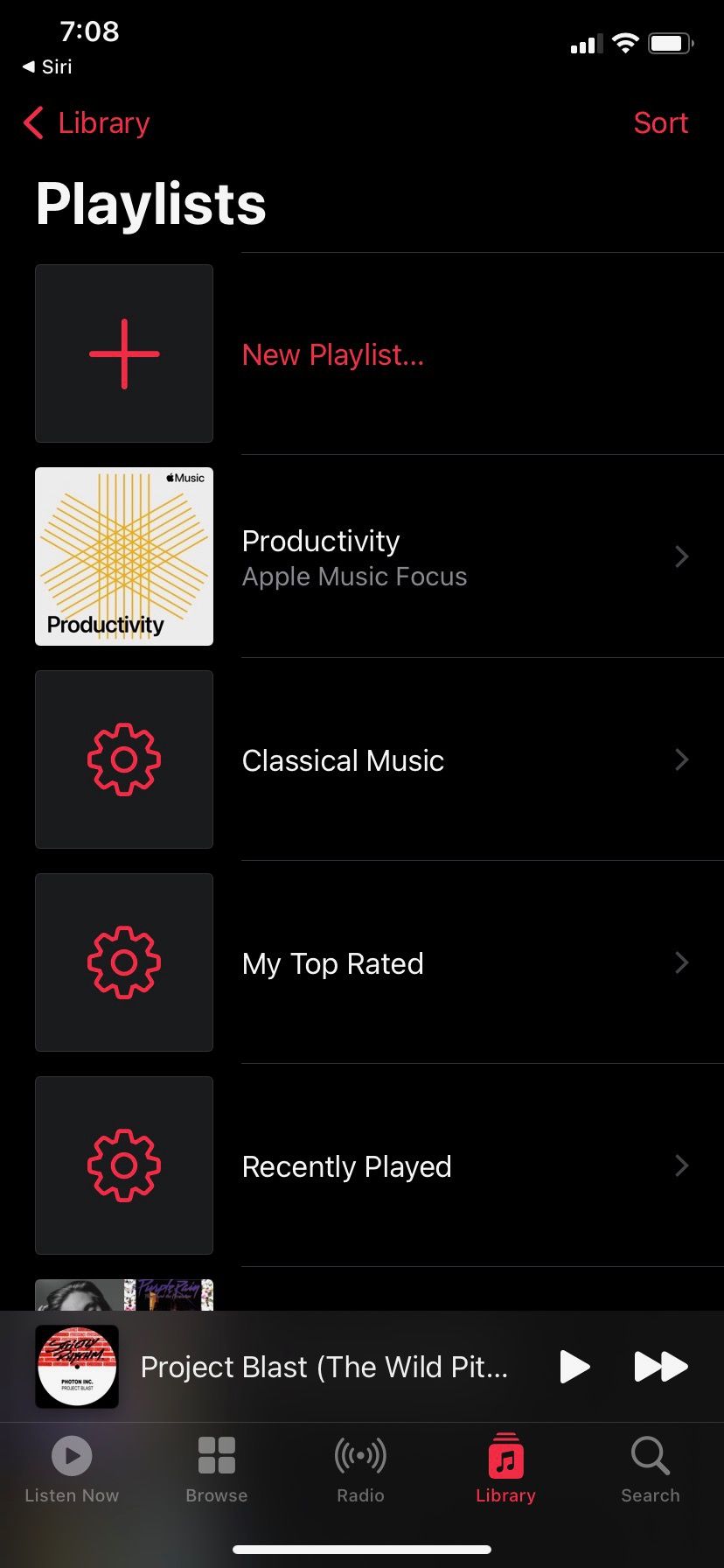In this screenshot of an Apple Music interface captured at 7:08, several key elements are displayed clearly. The top left corner shows the current time and beneath that, the word "Siri" with an arrow pointing left. Directly below it reads "Library" with another left-pointing arrow. On the top right, icons display a fully charged battery, Wi-Fi at full strength (four bars), and a mobile signal with three bars.

In the middle top section, the word "Playlist" is prominently displayed in bold, white text positioned above a vertical column of five neatly aligned square boxes. Each box contains different content: 

1. The first box features a plus symbol with the text "New Playlist..." on its right.
2. The second box labeled "Productivity" has a white backdrop and is marked with "music" in the top right, followed by "Productivity, Apple Music Focus."
3. The third box showcases an image of a gear with the label "Classical Music" beside it.
4. The fourth box, also with a gear icon, is titled "My Top Rated."
5. The fifth and final box is a gear icon labeled "Recently Played."

On the right side of "Library," towards the east portion of the image, there is a "Sort" option, indicating organizational tools for the displayed playlists.